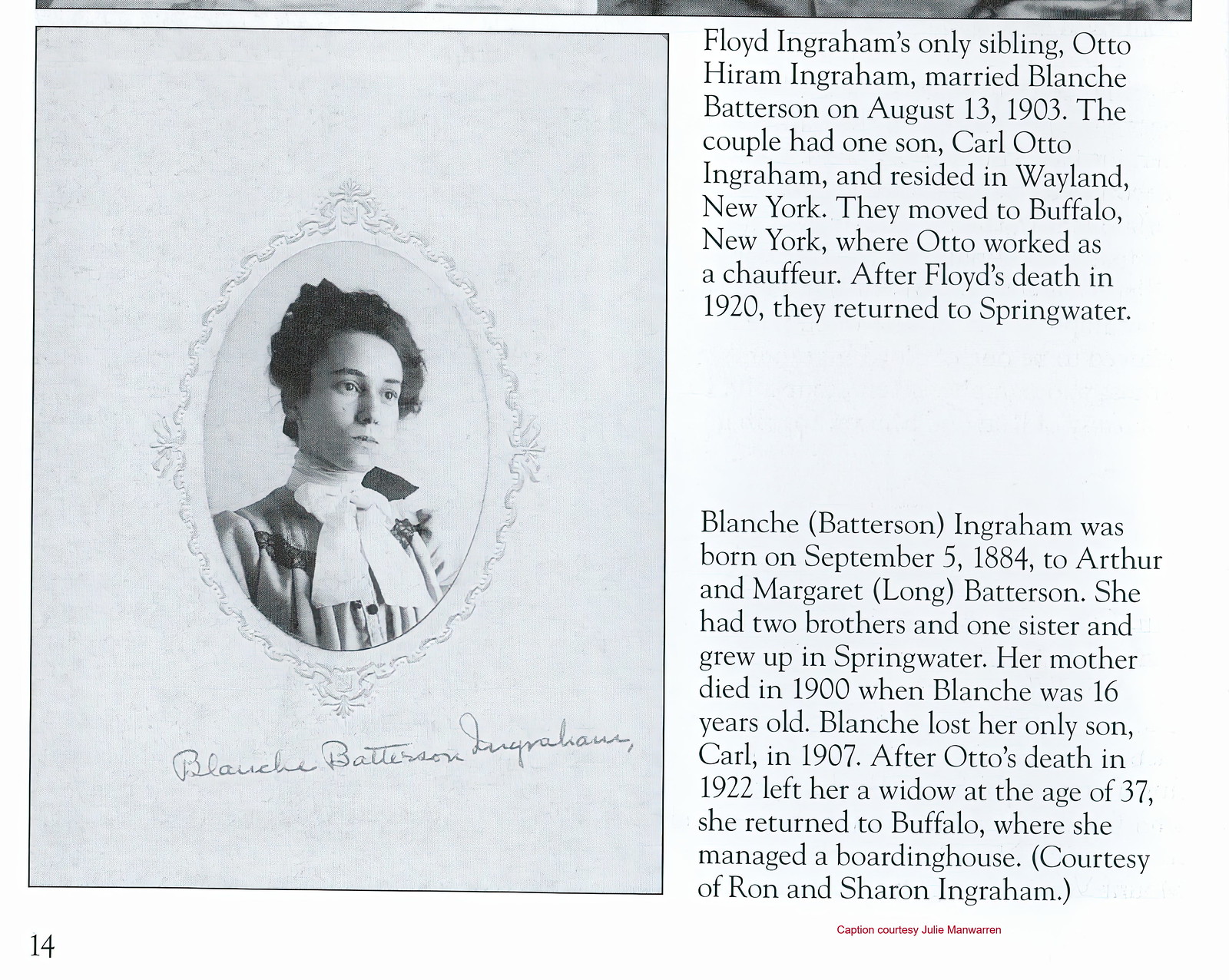The image displays a page from a book, characterized by a clean white background with the number 14 printed in black text at the bottom left corner. The left side of the page features an oval black-and-white portrait of a woman, facing towards her right, set against a gray background. The woman is elegantly dressed in a modest dress adorned with a neck scarf and buttons running up the front, with her hair styled upward into a bow. Below the portrait, the handwritten name "Blanche Batterson Ingraham" is inscribed in cursive. 

To the right of the portrait, there are two columns of text that provide detailed historical context. The text begins with the information that Floyd Ingraham's only sibling, Otto Hiram Ingraham, married Blanche Batterson on August 13, 1903. The couple had one son, Carl Otto Ingram, and initially resided in Wayland, New York before moving to Buffalo, New York, where Otto worked as a chauffeur. After the death of Floyd Ingraham in 1920, the family returned to Springwater. The text also reveals that Blanche Batterson was born on September 5, 1884, to Arthur and Margaret Batterson and had two brothers and one sister. Tragedy struck early in her life with her mother's death in 1900 when Blanche was just 16 years old. She later faced further sorrow when her only son, Carl, passed away in 1907. After Otto's death in 1922, which left her a widow at the age of 37, Blanche returned to Buffalo and managed a boarding house.